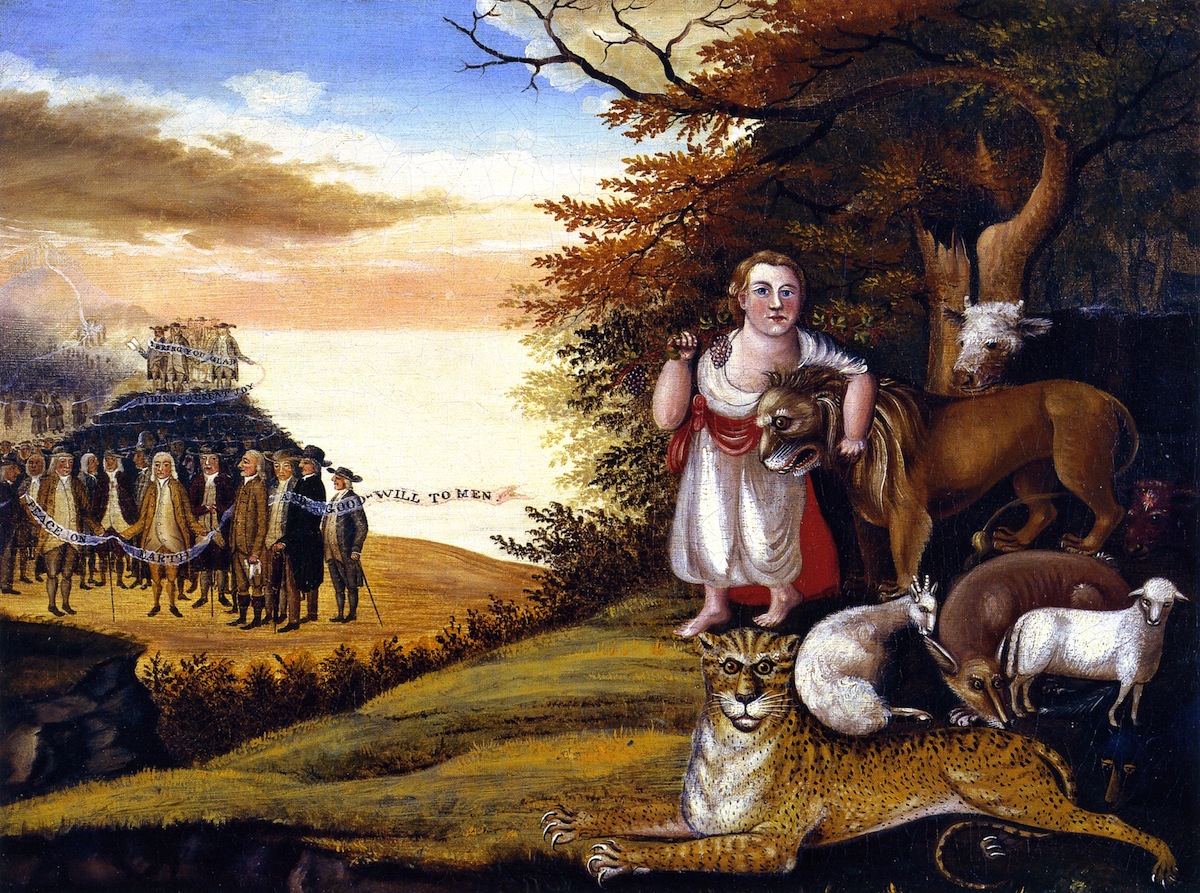This painting, titled "Peaceable Kingdom" by Hicks, is a vivid depiction of an outdoor scene set during the daytime in the folk art style, reflective of early American art. Dominating the right side, a woman or child wearing a white robe with a red belt, and possessing reddish hair, tenderly embraces a lion. In her other hand, she holds a bunch of grapes. She stands under the shade of a tree, with a cow beside the trunk. At her feet, a panther lies calmly, surrounded by sheep and goats. The ground beneath her is a yellowish hue.

On the left side of the painting, a group of men, possibly settlers or colonists resembling Quakers, gather in a semicircle around a central figure dressed in a long brown jacket. Many of these men wear traditional Quaker hats and some carry canes. The central figure holds a prominent banner that reads "Peace on Earth, Goodwill to Men." In the background, another group of similarly dressed men and more settlers can be seen, faintly sketched, also carrying a banner.

The setting features a contrasting landscape with blue skies accented by brownish, white, and peach-colored clouds. There is a glimpse of an ocean, and the entire scene is enveloped in a serene, pastoral atmosphere that underscores the painting's theme of harmonious coexistence among humans and animals alike.